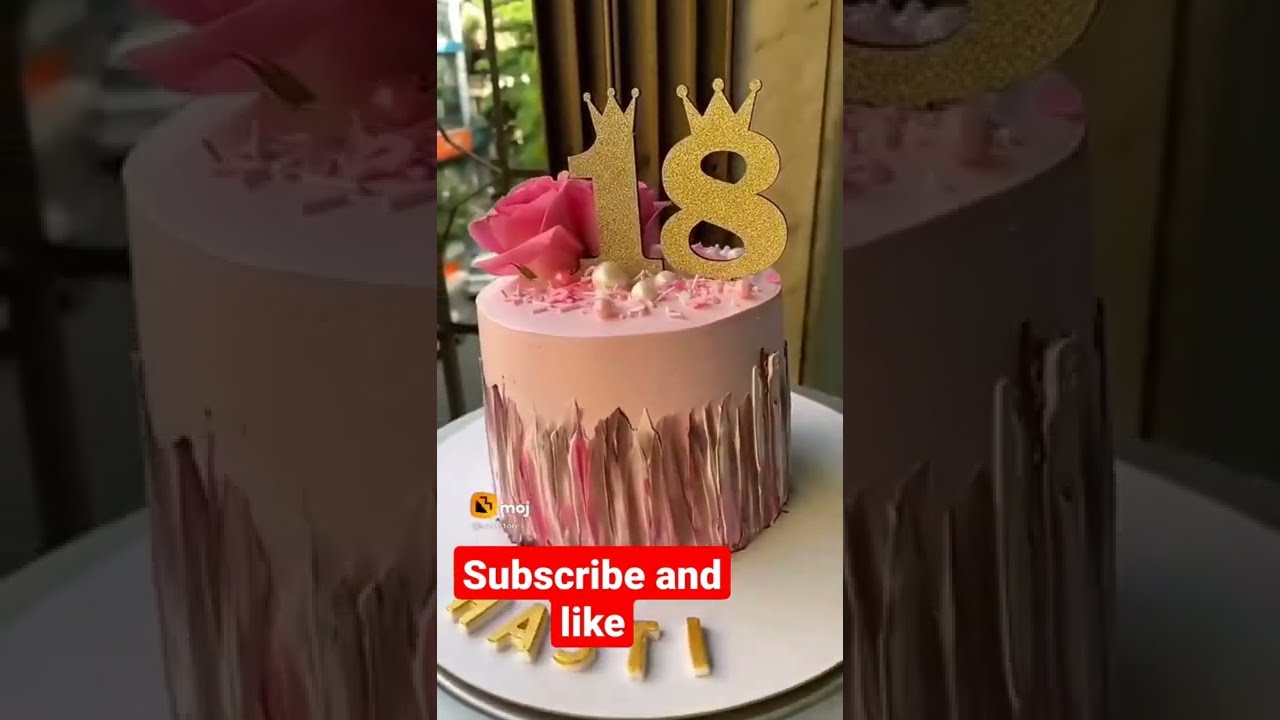This image is a screen grab from a TikTok or Instagram video, showcasing a highly decorated and professionally crafted 18th birthday cake. The cake itself is a perfect, cylindrical shape, with a flawlessly smooth buttercream icing of soft pink color. The bottom of the cake features an abstract design resembling overlapping feather shapes, done in darker pink and brownish-purplish tones, extending upwards. The top of the cake is adorned with pink and white sprinkles, edible pearls in various shades of pink and white, and two real pink roses. Crowning the cake is a glittering gold cutout of the number "18," each number topped with a crown, situated right in front of one of the roses. In the background, natural light filters through a window. A prominent red button with white text reading "subscribe and like" is visible at the bottom, indicating this image captures a moment from the end of a cake decorating video. The visual composition involves both a zoomed-out and a zoomed-in version of the cake, the latter with a darker filter, illustrating the intricate details and professional finish of the decorated cake.